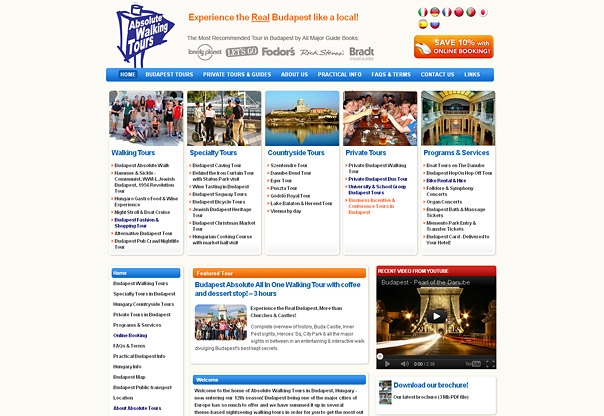A vibrant webpage promoting Budapest walking tours is highlighted with striking orange and white text. The header reads "Experience the Real Budapest Like a Local," with "real" underlined for emphasis. A compelling offer to "Save 10% with Online Booking" stands out in white text on an orange rectangle. The navigation bar, adorned in blue, features tabs: "Home" (selected in dark blue and white), "Tours," "Private Tours," "Guides," "About Us," "Practical Info," "FAQs," "Contact Us," and "Links."

The main content is divided into five sections: "Walking Tours," "Specialty Tours," "Countryside Tours," "Private Tours," and "Programs and Services," all written in blue. The "Home" section lists a featured tour titled "Budapest Absolute All-in-One Walking Tour with Coffee and Dessert Stop (3 hours)." Next to the welcome text is a recent YouTube video with a play symbol at its center, ready to offer visitors a preview of the tour experience.